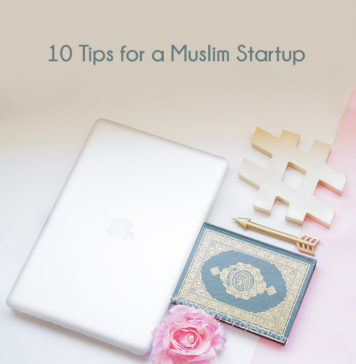The image shows a meticulously arranged flat lay with a predominantly light pink background, gradually transitioning into white. At the top, in clear text, it reads, "10 Tips for a Muslim Startup." Central to the composition is a sleek silver laptop with an unmistakable Apple logo. On the surface, a single pink rose adds a touch of elegance next to a distinct arrow-shaped object, likely a decorative ink pen. A small card or notebook, bearing what appears to be a Muslim emblem, lies nearby, though its cover is devoid of any visible text. Additionally, a silver hashtag or pound symbol is positioned close to the pen, contributing to the thematic decor. The entire setup rests on what seems to be a clean, minimalist table, contributing hues of pink, blue, silver, and white to the scene's harmonious color palette.